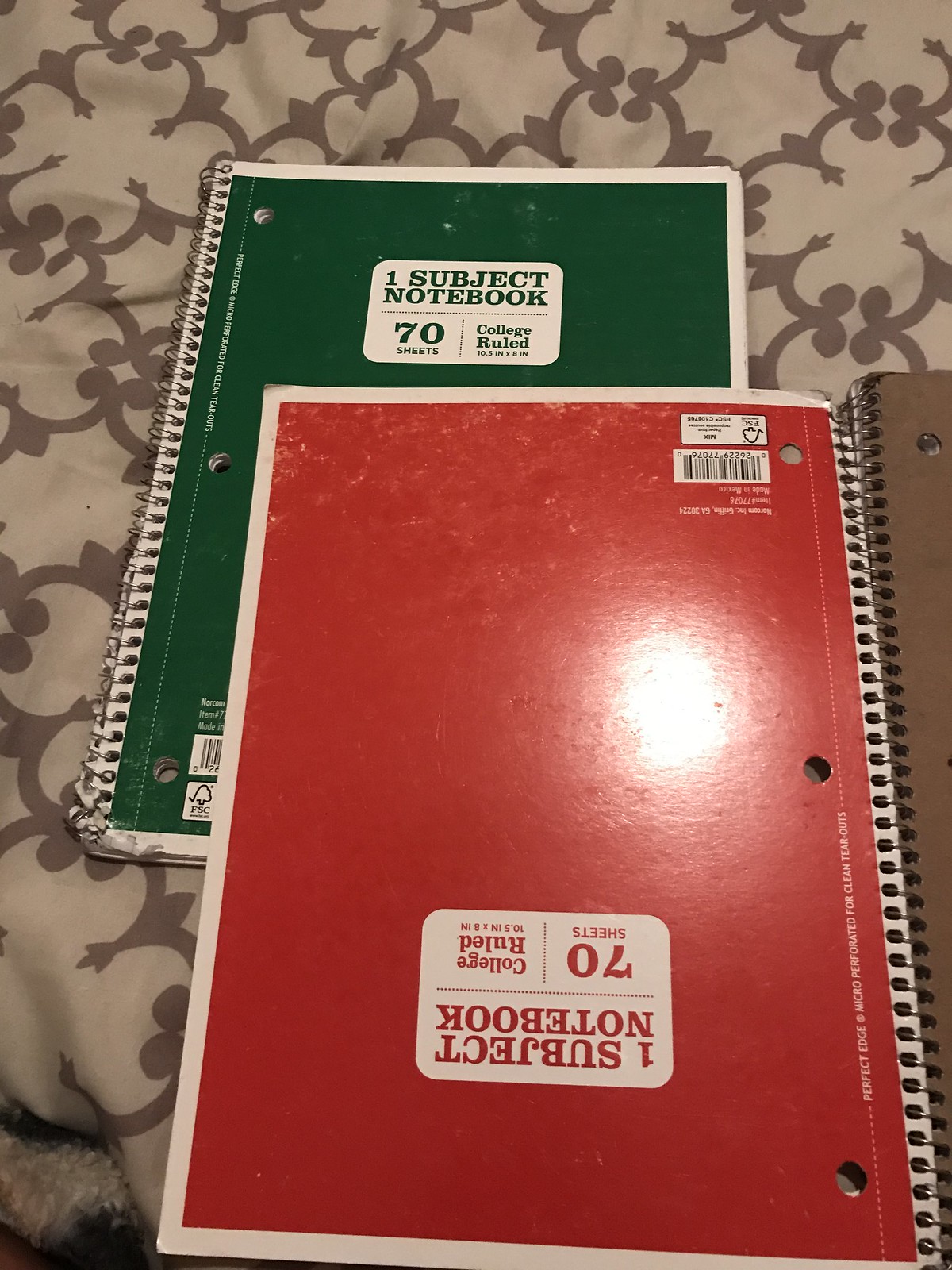This photograph captures an indoor scene showcasing two spiral-bound notebooks, one atop the other, sitting on a surface with an off-white, cream, and brown floral-patterned material, possibly a tablecloth or comforter. The bottom notebook is green and positioned correctly, displaying a white rectangular label at the upper center that reads "One Subject Notebook, 70 Sheets, College Ruled." On top of it lies a red notebook, turned upside down with its spiral binding to the right. Both notebooks appear slightly worn, with faded covers and minor damage to the binding, suggesting they've been used. A hint of a third spiral notebook is visible at the edge of the image, too indistinct to identify. The photo is illuminated by a flash, evident from the glare on the red notebook's cover.